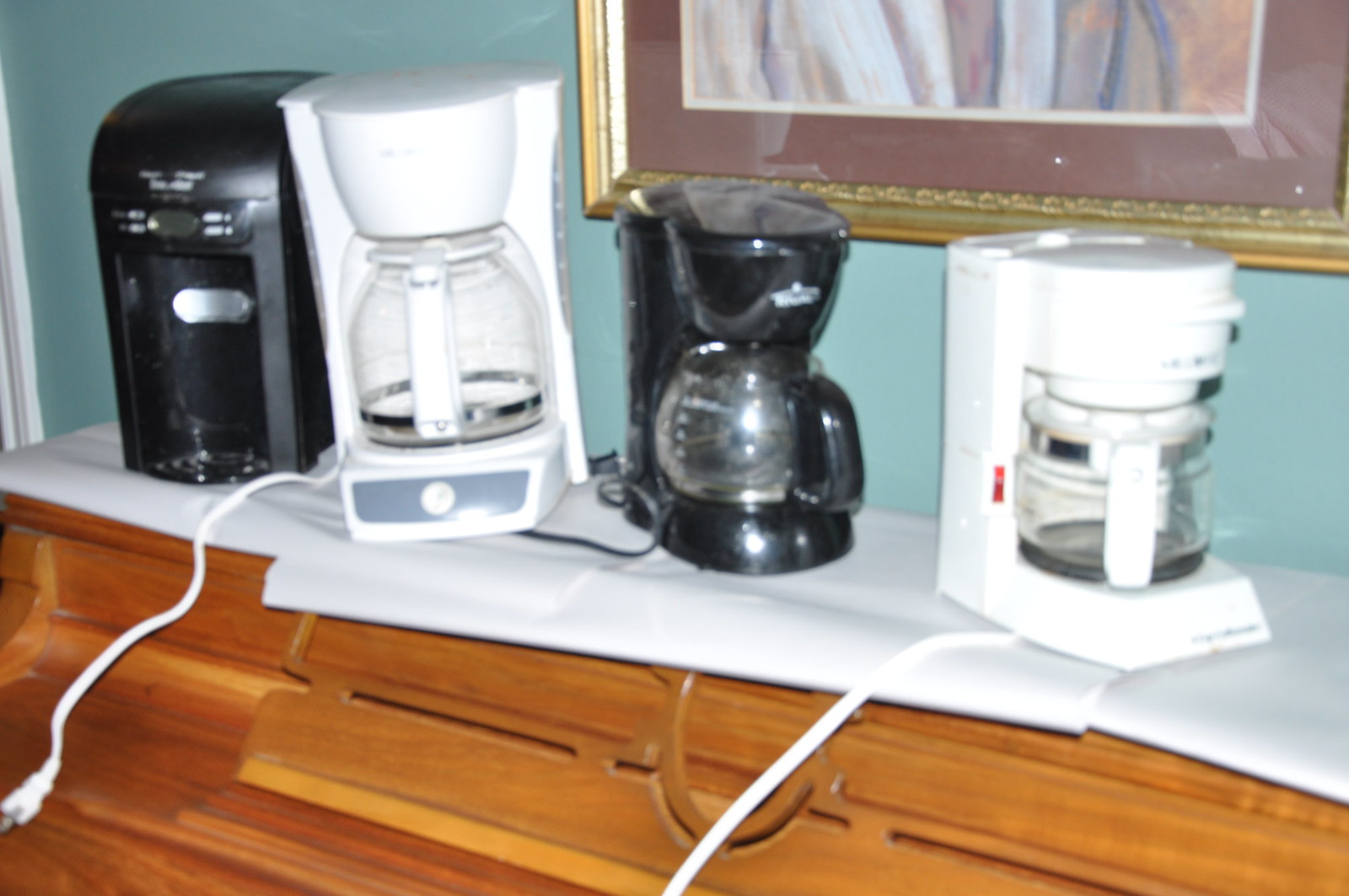This photograph captures a row of four coffee makers displayed atop a shelf of drawers made of blonde wood. The shelf is lined with white paper, providing a clean surface for the coffee makers. Arranged in an alternating pattern, the coffee makers are positioned as follows: a solid black machine on the far left, followed by a white one, another black one, and finally a white one on the far right. Each coffee maker features a clear glass carafe, except for the first black coffee maker, which is a more modern design allowing for direct dispensing into a cup with the press of a button. The image quality is grainy and slightly blurry, suggesting it might be an old photograph. The backdrop is an aqua blue painted wall, adorned with a framed portrait just above the coffee makers, of which only the lower part with brown matting and golden frame is visible. The drawers below the shelf are long and extendable, contributing to a functional yet aesthetically pleasing setup.